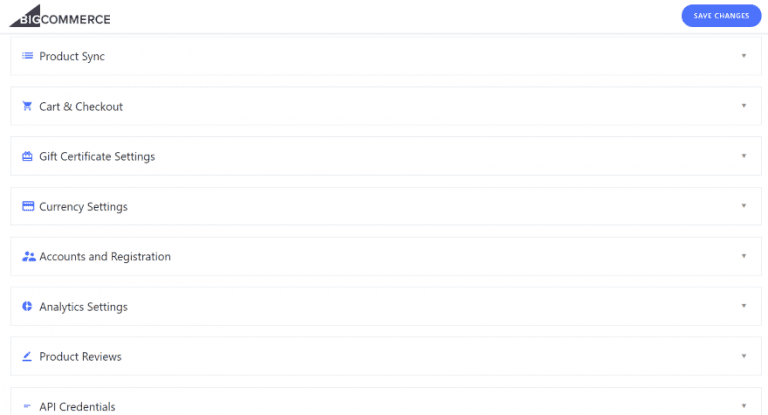This is a detailed screenshot of a settings or options page on an e-commerce website. In the top left corner, there is a logo for "BigCommerce," styled in thick black font with an inverted triangle beneath the word "Big" in "BigCommerce". To the right of the logo, there's a prominent blue button labeled "Save Changes" in white font.

Below these elements, the page is organized into various sections, each representing different settings options:

1. **Product Sync**
   - A row titled "Product Sync" is displayed prominently at the top.

2. **Cart & Checkout**
   - A section for "Cart & Checkout" with a cart icon on the left and a drop-down box icon on the right.

3. **Gift Certificate Settings**
   - This row features a blue gift box icon on the left and a drop-down box on the right.

4. **Currency Settings**
   - Displayed with a blue credit card icon to the left and a drop-down box to the right.

5. **Accounts & Registration**
   - This section is marked by a blue people icon on the left with a corresponding drop-down box on the right.

6. **Analytics Settings**
   - Highlighted with a circular icon on the left, paired with a drop-down box on the right.

7. **Product Reviews**
   - This row includes a small pencil and paper icon on the left and a drop-down box on the right.

8. **API Credentials**
   - Identified with a tiny blue key icon on the left and a drop-down box on the right.

The overall design is clean and intuitive, with easy access to various settings through drop-down boxes, accompanied by relevant icons for quick recognition.